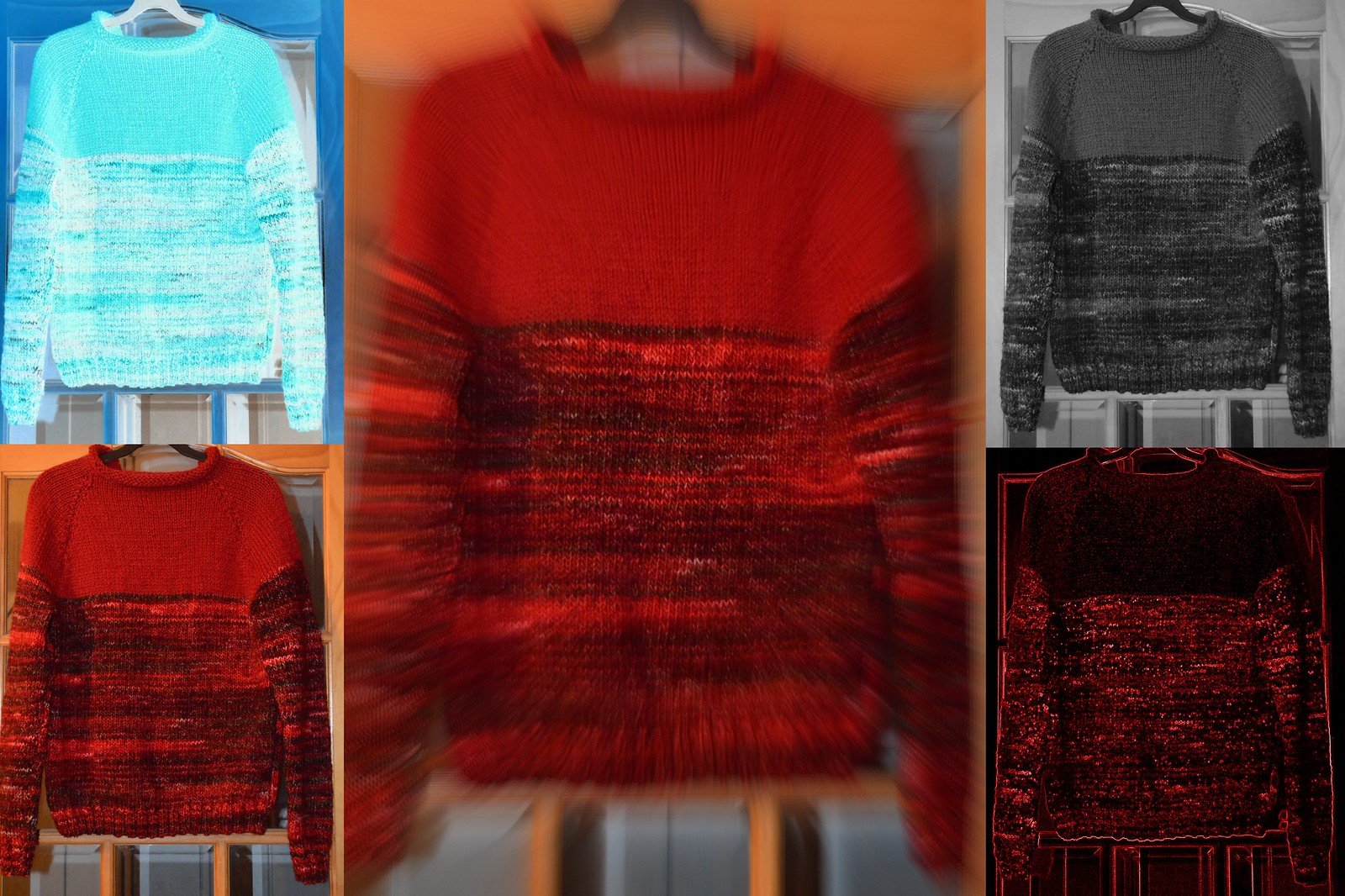This image features a collage of five photos showcasing a single sweater, each with distinct visual effects and color variations. The first photo on the top left presents a light blue sweater with subtle white stripes, hanging on a wooden coat hanger against a blue wooden frame backdrop. Directly below it, there’s another photo showing the same sweater design, but it’s red with black striping. The middle image magnifies this red and black sweater but is heavily blurred, creating a disorienting, almost psychedelic effect. To the right, the top photo displays the red and black sweater in a black-and-white filter, rendering it in shades of gray. The bottom-right photo inverts the colors of the sweater, making the red areas appear black and the black areas appear red, giving it a shadowy, darker appearance. All the sweaters are hung neatly on coat hangers, emphasizing their consistent style despite varying visual treatments.